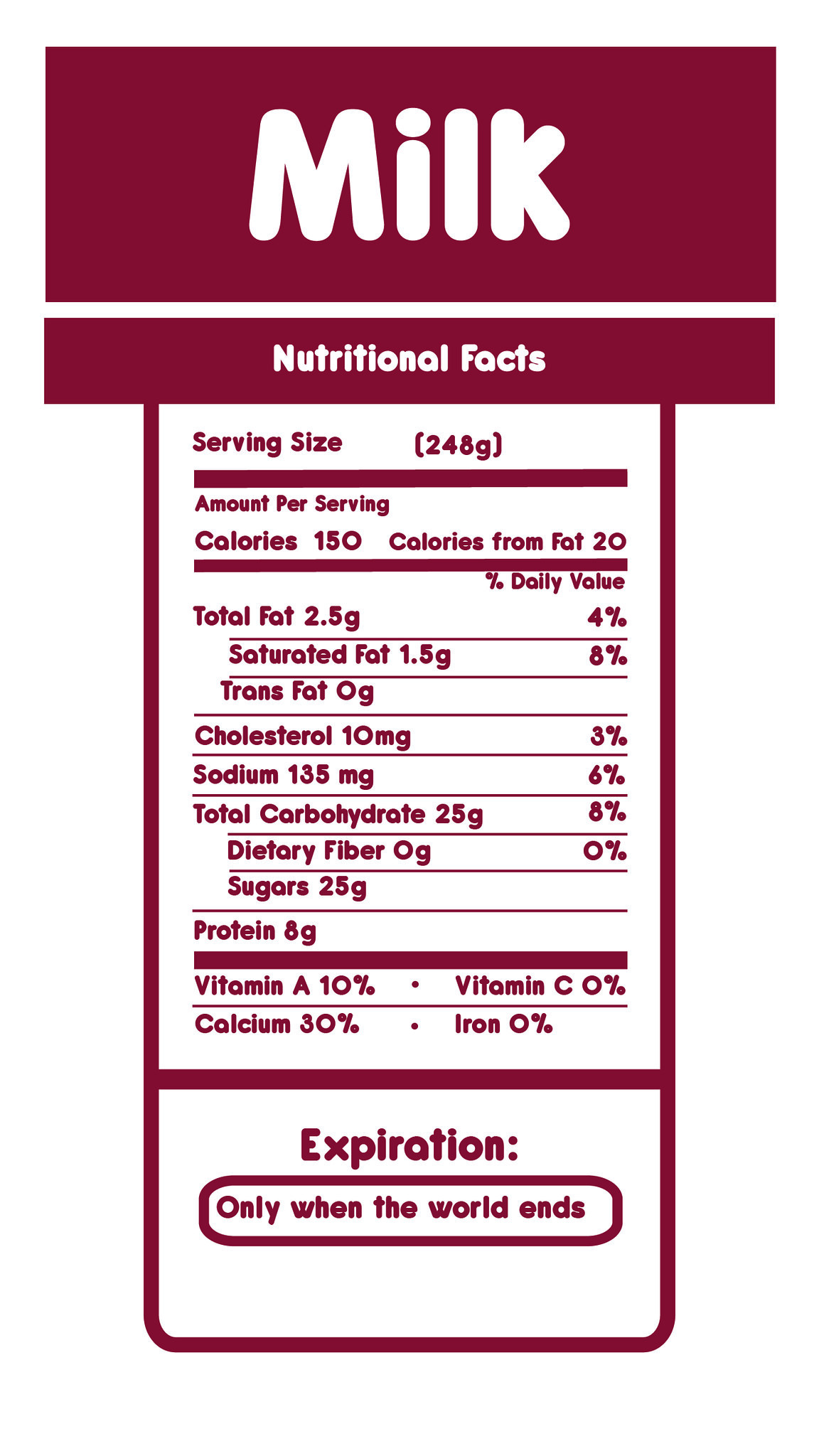This close-up image captures an informational graphic titled "Nutritional Facts for Milk." At the top of the graphic, the word "Milk" is prominently displayed in bold white text, followed by the phrase "Nutritional Facts," also in white, both centered against a burgundy background. Below this header, detailed nutritional information is provided in burgundy text on a contrasting white background, making the data easily readable. Notably, at the very bottom of the graphic, there is a playful element: an oval containing the humorous statement, "Expiration only when the world ends." The overall design is minimalist, featuring a transparent background with no border, adhering to a strict burgundy and white color scheme.